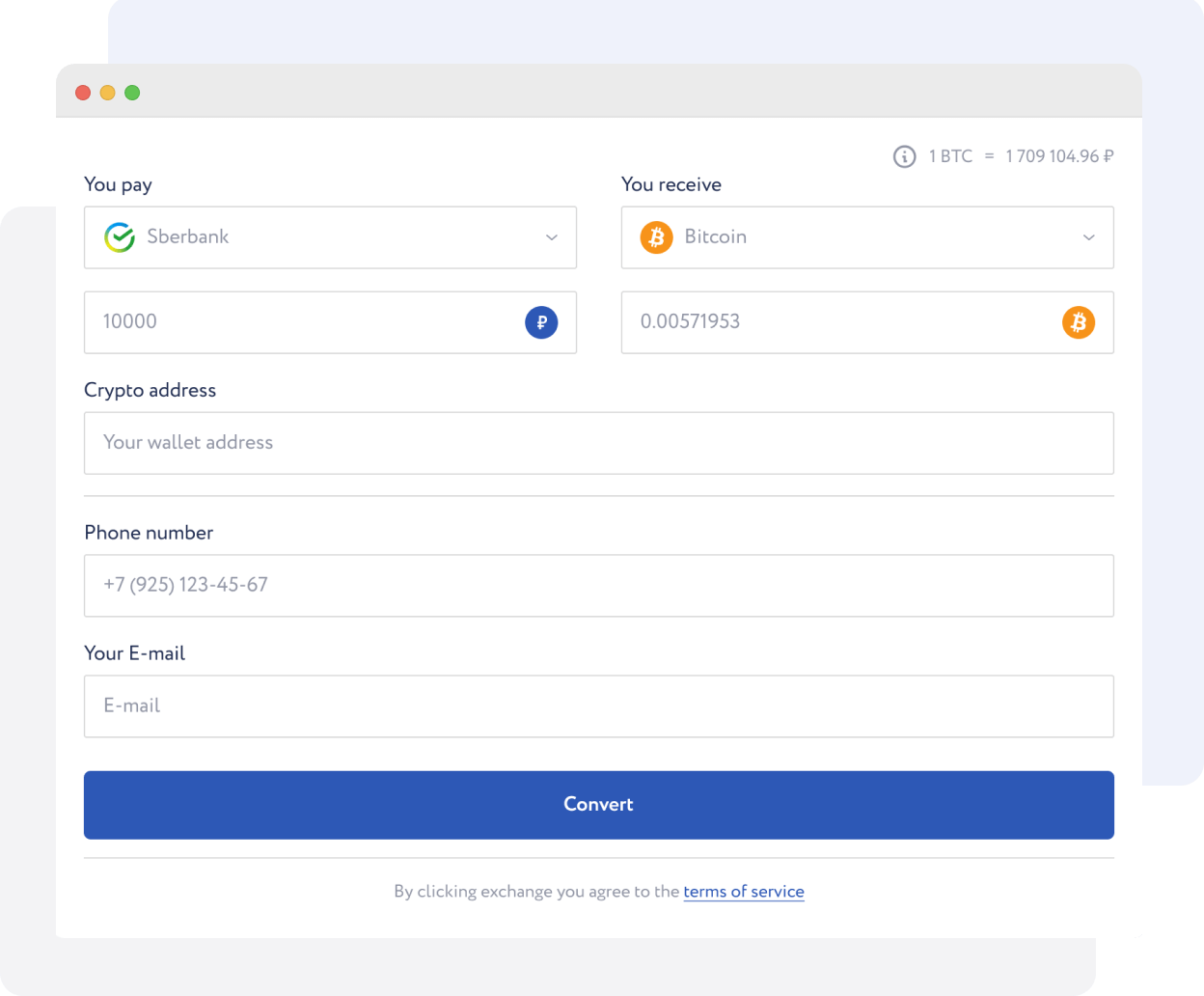At the top of the image, there is a section featuring a light blue area followed by a light purple area. On the left side of these sections, there are three circles: a red circle, an orange circle, and a green circle. Below these visuals, the background turns white and displays the text "You Pay."

Underneath "You Pay," there is a text box accompanied by a drop-down button labeled "SBER bank." Below this dropdown, another text box displays the amount "10,000." Adjacent to this is a blue circle with the letter "P" in the middle. Beneath this circle, a label reads "Crypto Address," followed by a text box prompting for "Your Wallet Address." Continuing downward, there is a label for "Phone Number" followed by a text box pre-filled with "+7 925 123-45-67." Further down, there is the label "Your Email," accompanied by a text box labeled "Email."

In the top right corner of the image, the text reads "You Receive," with a box displaying an orange circle and a capital "B" in the center, indicating Bitcoin. Below this, another box with the same orange circle and "B" symbol shows the value "0.00571953."